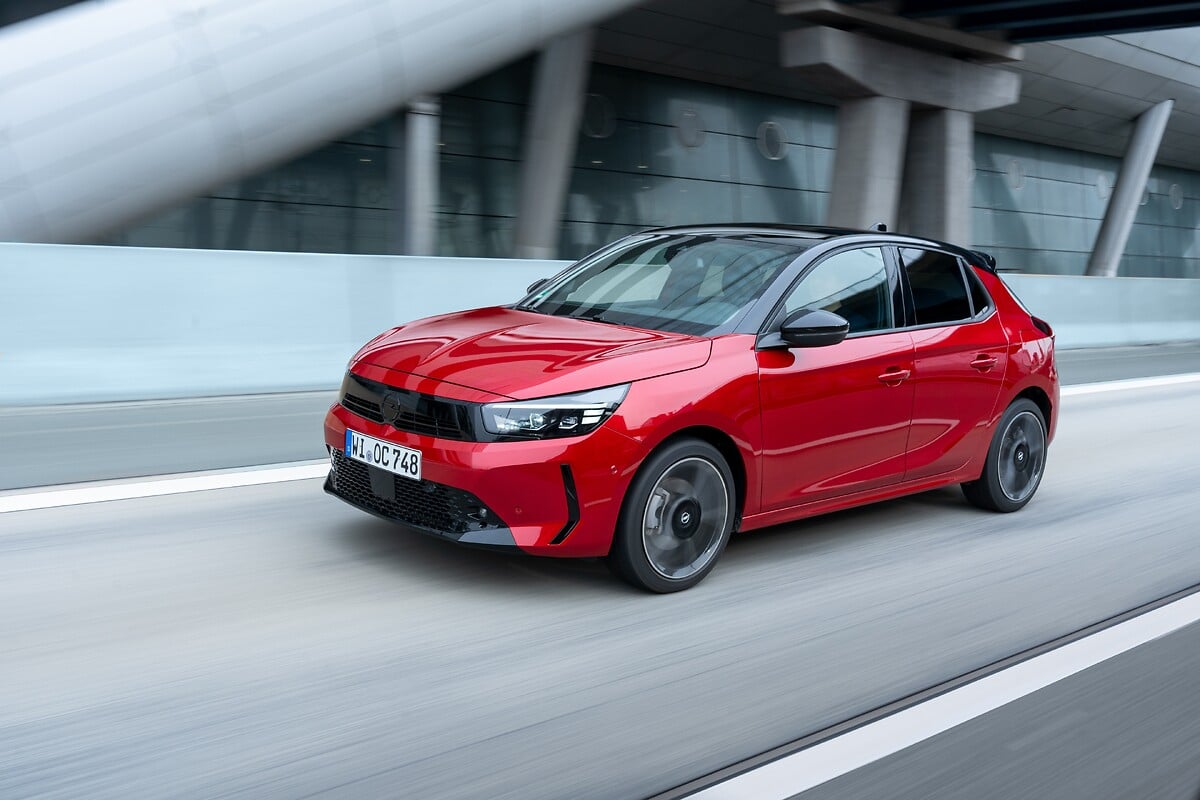A vibrant red sedan is captured mid-motion, driving from right to left on a paved road marked by white lane dividers and a dark gray center strip. The vehicle is adorned with black windows, a black grille with a small slit underneath the headlights, and is accented by black wheels with silver rims. The front of the car, slightly angled toward the camera, reveals its European-style license plate with visible characters "OC748." The scene is set against an urban backdrop, dominated by a large concrete structure supported by rectangular pillars. In the background, a diagonal pillar cuts across the top left corner of the image, adding a dynamic architectural element. A continuous gray barrier runs parallel to the road, separating the vehicle from the imposing building behind it. The road, devoid of other cars, emphasizes the focus on the speeding red car, which remains sharply in focus while the background appears muted in motion blur. The image captures the essence of urban travel under a sprawling concrete overpass.